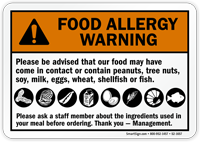The image showcases a rectangular label with rounded corners set against a solid white background. This sticker features a neat design with a thin black border dividing the interior into two sections. The top section, approximately one-third of the label, has an orange banner background with black text that states, "Food Allergy Warning," accompanied by a black triangle icon containing an orange exclamation mark. Below this banner, the white section of the label conveys an advisory in black text: "Please be advised that our food may have come in contact with or contain peanuts, tree nuts, soy, milk, eggs, wheat, shellfish, or fish." This section also includes respective icons for each allergen such as peanuts, wheat, shrimp, and fish. The label concludes with the message, "Please ask a staff member about the ingredients used in your meal before ordering. Thank you, Management."